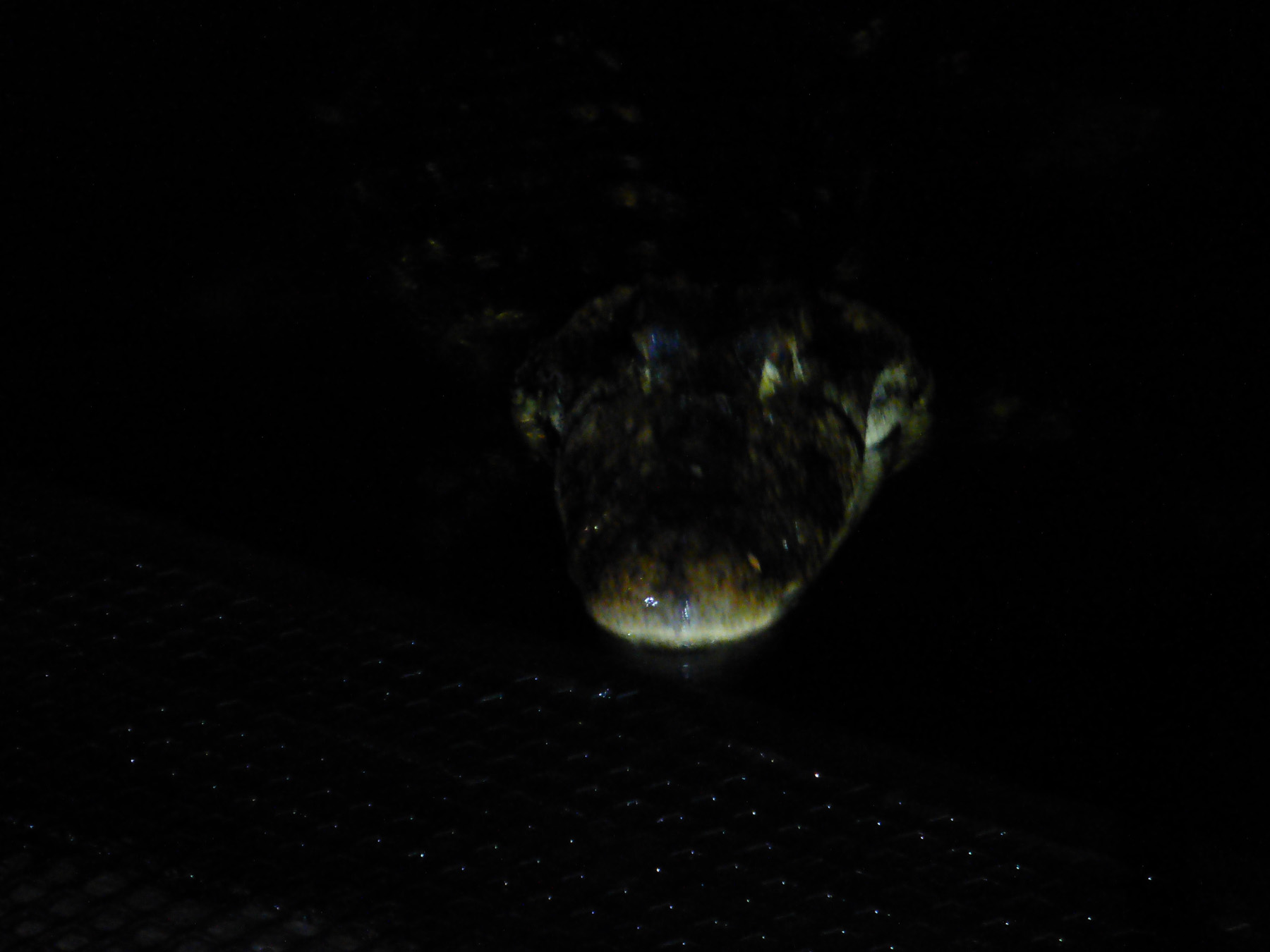In the image, taken at night, the scene is enveloped in almost complete darkness, with a pitch-black background. At the bottom, a black metal platform with a multitude of holes, resembling a drainage grate, stretches from the mid-left down to the lower right corner. Emerging from the water at the center, slightly to the right, is the head of a reptile, likely an alligator or crocodile. The animal's snout, which is facing slightly towards the left, has a tan tip. Its eyes, located in the middle of its head, reflect a hint of yellow in the dim light. The reptile's head displays a range of colors, from greenish hues to dark almost black areas, with the surface of the water subtly surrounding it. Around the creature, tiny white specks are visible, adding a faint texture to the otherwise inky backdrop.